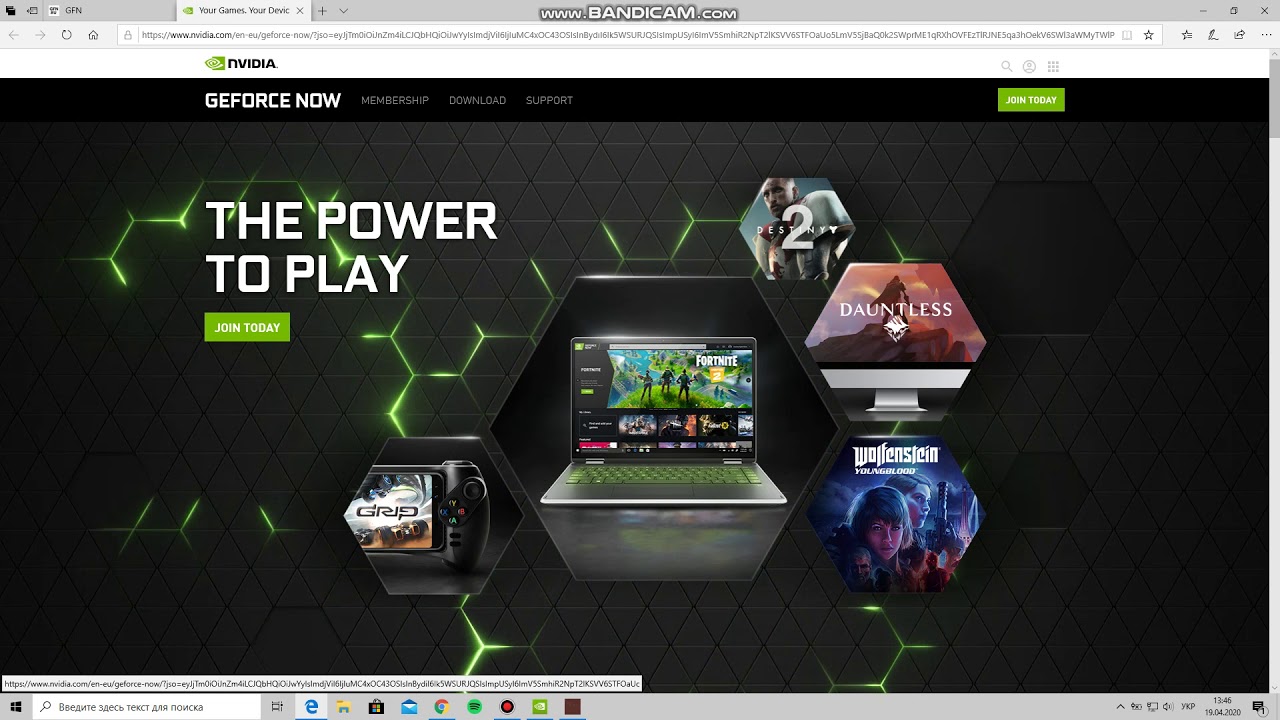This image is a screenshot of a Windows computer screen displaying the Edge browser in widescreen mode. At the very top is a thin gray banner, featuring the URL "www.bandicam.com" prominently in the center. In the upper left corner, there are several open browser tabs, including a CNN tab and another tab with a green icon, indicating it is the NVIDIA site.

Beneath the URL banner is the browser's toolbar, containing buttons for navigation such as forward, back, home, and refresh. The URL input field within this bar is populated with a lengthy URL, though it is too small to be legible.

Below this toolbar is another gray banner labeled "NVIDIA," highlighted by the green NVIDIA icon positioned towards the left but not quite at the edge. To the right, there are three additional icons, placed near but not at the far right edge of the banner.

The main portion of the screen showcases the black-themed NVIDIA website, with "GeForce Now" displayed in bold white text at the top-center. Adjacent to this text is a section with additional content in dark colors, rendering it difficult to decipher. There's a green button in the upper-right corner, the text of which is unreadable.

Further down, the website features images of a computer surrounded by octagonal frames showcasing popular games such as Dauntless, Wolfenstein, and Destiny 2 on the right side. Text on the left side reads "The power to play," accompanied by a green "Join Today" button.

The very bottom of the screenshot includes a gray banner comprising the Windows taskbar, which features the Start button, search bar, quick access icons, and the system tray on the lower right.